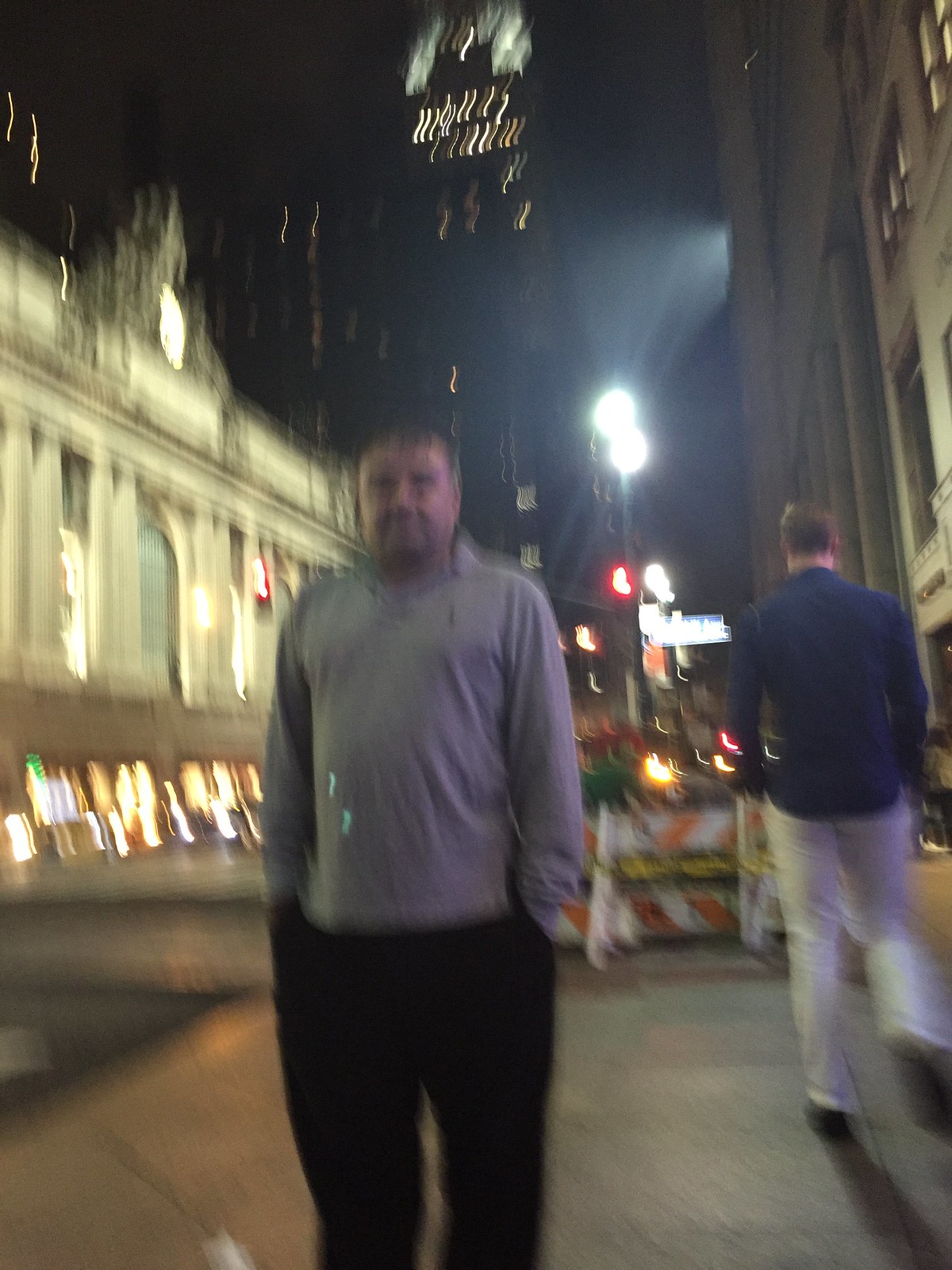Captured in the heart of downtown at night, this vibrant city scene is illuminated by the glow of streetlights and the headlights of passing cars. The bustling street is flanked by a prominent building on one side and a sidewalk on the other. A caution sign suggests ongoing construction, subtly guiding pedestrians around the area. On the sidewalk, two men are present: one is facing the camera, dressed in black pants and a long-sleeved gray shirt, while the other, with his back to the lens, is wearing a long-sleeved blue shirt and white pants. The interplay of lights and shadows adds a dynamic energy to the nocturnal urban landscape.